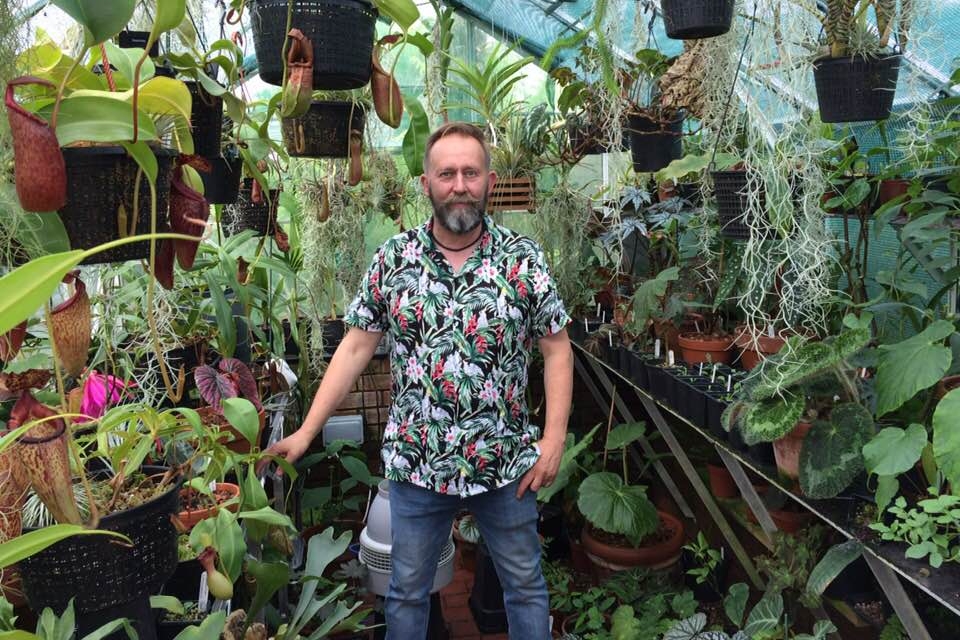The photograph captures a middle-aged man standing in the center of a bustling greenhouse. He sports a Hawaiian-style floral shirt in black, green, and white, paired with blue jeans. His short brown hair is tinged with gray, and he has a gray-speckled beard and mustache. The greenhouse, bathed in daylight thanks to its glass ceiling and walls, is filled with a diverse array of plants. There are potted plants all around, some perched on tables, some on the floor, and many hanging from the ceiling. The flora includes hanging plants, palm-like trees, begonias, vines, corpse flowers, and various blooming pots. A brown woven basket filled with plants is visible on the left side of the image. The man stands confidently, looking directly at the camera, amidst the verdant abundance.